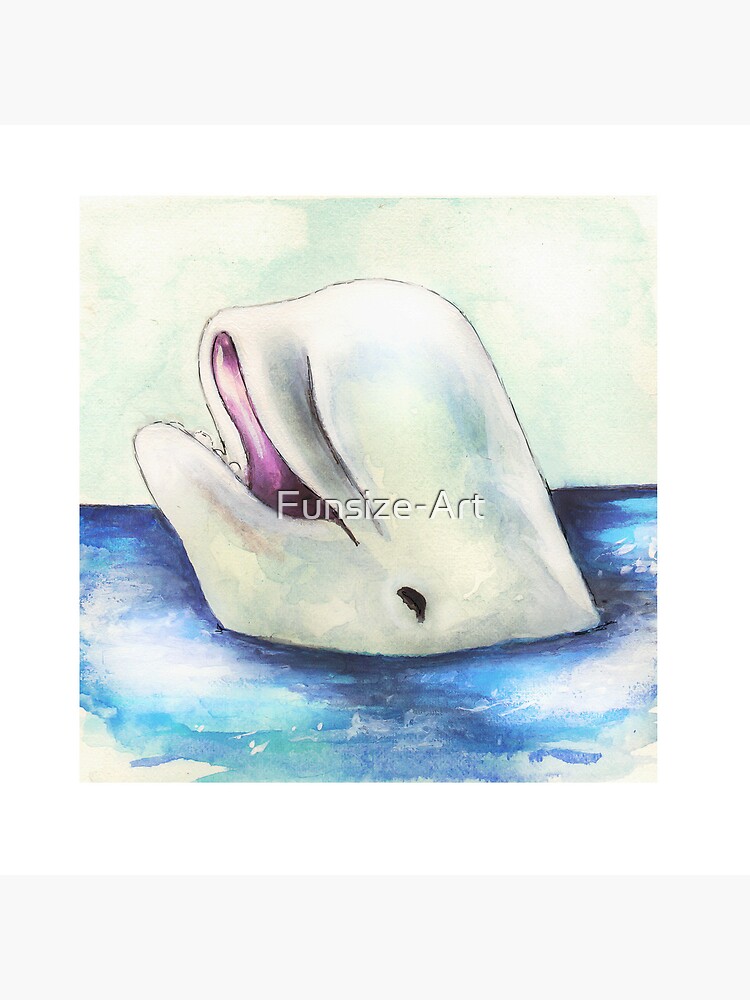The image is a whimsical drawing titled "Fun Size Art," prominently displayed in white letters across the center. The background features a delicate, pale blue sky dotted with soft white clouds. Beneath this serene sky lies the blue ocean, characterized by splashes of white, suggesting a gentle movement. At the forefront of the scene is a playful illustration of a large white whale. The whale's mouth is agape, revealing a purplish interior and glimpses of its white teeth. One expressive eye gives the impression of the whale smiling, radiating a sense of happiness and contentment. The ocean water surrounding the whale displays a harmonious blend of white, light blue, and darker blue hues, capturing the dynamic yet tranquil essence of the sea.